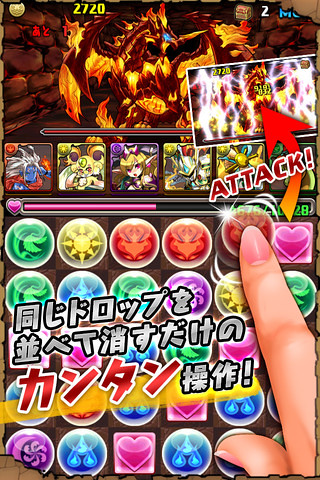This is a digitally rendered, highly colorful poster for a cartoon-like mobile video game. Central to the image is a detailed depiction of a Caucasian woman's hand with peach-colored skin, darker accents around the knuckles, and fingernails painted pink with hot pink edges and white fingertips. Her pointer finger is pressing a red, circular button labeled "attack" in bold red letters with a white border.

Surrounding this hand are various colored buttons featuring different symbols, including red, yellow, green, blue, and purple circles, as well as pink squares with hearts. These buttons are likely part of a match-3 style game mechanic. There's an array of Asian symbols and lettering in red, gray, and white, some of which accompany vibrant graphics such as a swish of orange and yellow around gray text with an exclamation point.

At the top of the image, there's a dragon-like creature with a red body and orange, flame-like wings, possibly indicating an in-game character. Accompanying the dragon is a number displayed in yellow, reading 2720, suggesting points earned or a score. Additionally, a treasure chest marked with the number 2 and an elf-like character with blonde hair and pink eyes are visible, enhancing the game's fantasy theme.

Overall, the poster showcases the game's dynamic and vibrant interface, promising an engaging and visually striking gameplay experience.